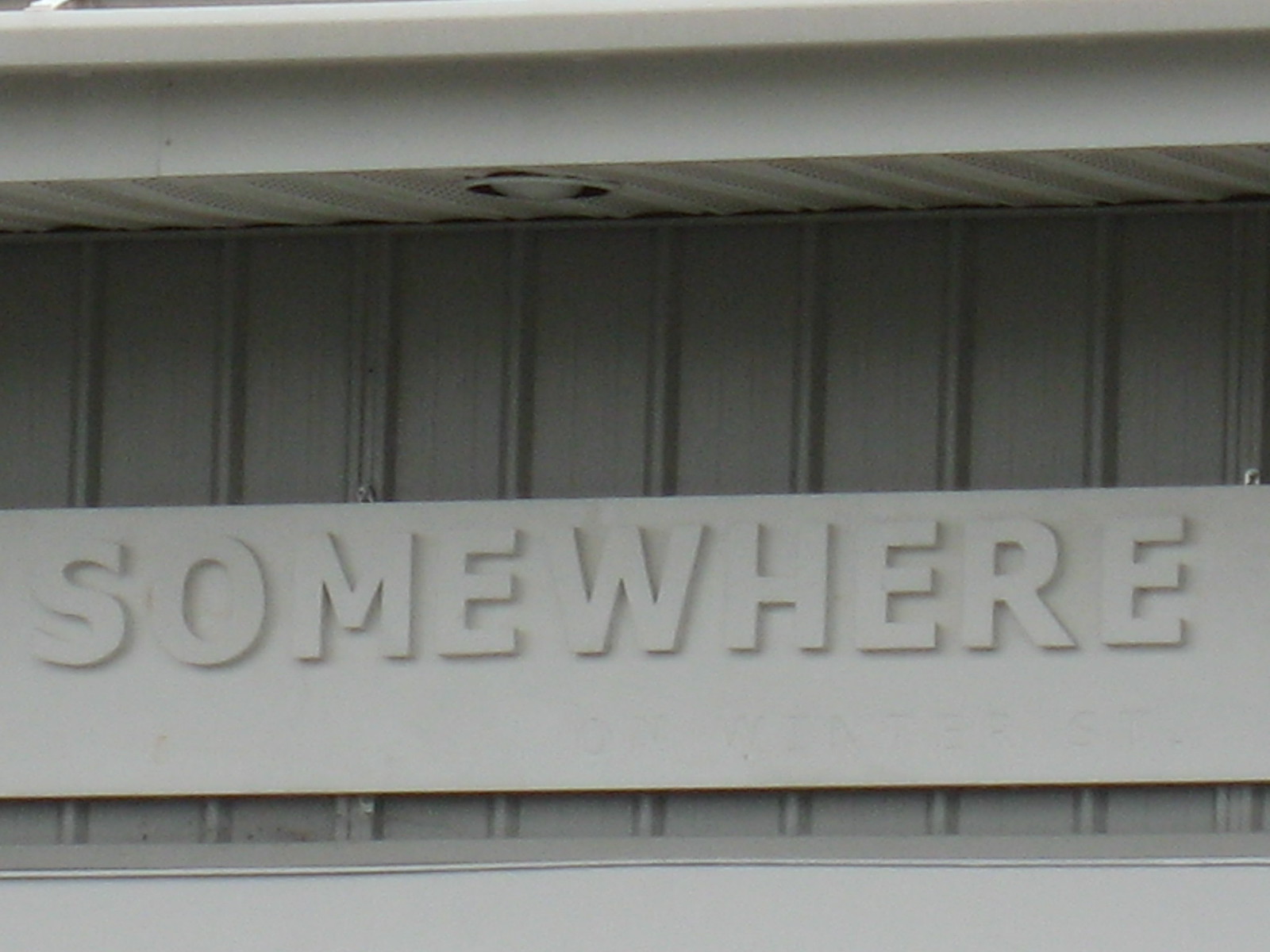This monochromatic photo captures an architectural section of a building, rendered in various shades of gray. At the top, a light gray overhang extends outward, casting a subtle shadow over the area beneath it. Below the overhang, there is a vented section, which features a circular light fixture prominently displayed in its center. The wall behind consists of vertical siding that varies in tones of gray, creating a textured backdrop. 

A light gray horizontal sign, emblazoned with the word "SOMEWHERE" in bold, 3D capital letters, is prominently attached to the wall. The 3D effect of the text is highlighted by the shadows cast by each letter. Beneath this sign, the vertical siding continues briefly, before giving way to an additional horizontal line of siding at the bottom of the image. The careful interplay of light, shadow, and varying shades of gray creates a compelling and detailed study of architectural elements.